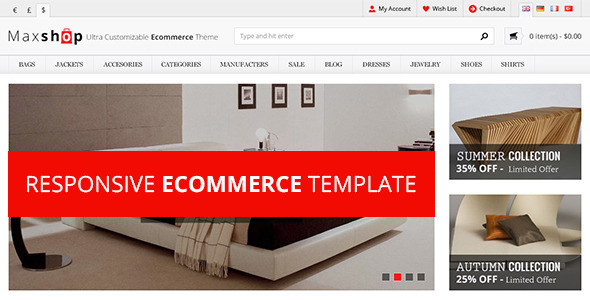This image showcases a horizontally-oriented web page, designed for access via computer or smart device. At the top, a long gray rectangular navigation bar spans the width of the page. On the upper left section of this bar, there are selectable currency options, with the dollar currently chosen. On the upper right, a series of icons enhance user experience: an account icon, a heart icon for the wish list, a checkout icon, and additional clickable options that appear to be country flags or similar symbols.

Further to the left, the web page is branded with "Mac Shop, Ultra Customizable E-commerce Theme." Adjacent to this, a white search bar invites users to "Type and hit enter," accompanied by a magnifying glass icon and a shopping cart icon displaying "0 items for $0."

A horizontal line demarcates the next section, which features a navigation menu listing clickable categories: Bags, Jackets, Accessories, Categories, Manufacturers, Sale, Blog, Dresses, Jewelry, Shoes, and Shirts. Despite appearing somewhat blurry, these words guide visitors to various product segments.

Central to the page is an image resembling a bedroom setting, with visible carpet, bed frames, and wall decor. Superimposed on this image is a thick red rectangular box containing the text "Responsive E-commerce Template" in white. This image, labeled as picture number two, indicates that users can scroll through further images.

On the right-hand side, promotional banners draw attention: one for the "Summer Collection" offering 35% off in a limited-time offer, and another for the "Autumn Collection" at 25% off, also presented as a limited offer. Each banner is accompanied by a relevant image.